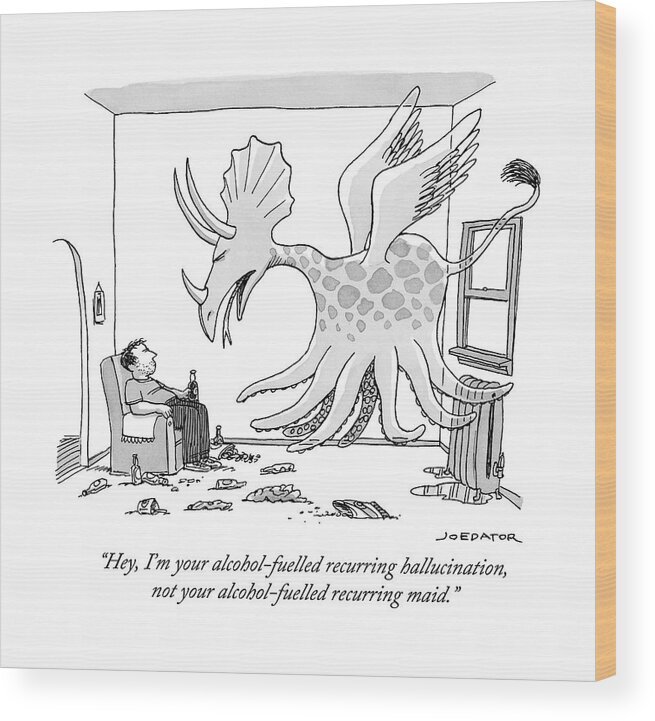This detailed comic-style drawing depicts a disheveled, slightly overweight man with scruffy facial hair lounging in a recliner, holding a drink in his untidy apartment. Scattered around him are chip bags, beer bottles, pop cans, and various other trash. The room includes a leaking radiator below a window, a doorway, and a single picture hanging above his chair. Floating above the man is a bizarre creature with features combining those of a triceratops, giraffe, octopus, and dragon, complete with wings and a snake-like tongue. The creature speaks, saying, "Hey, I'm your alcohol fueled recurring hallucination, not your alcohol fueled recurring maid." The artwork, painted over wood with visible wood grain and white overlay, emphasizes the dire straits of the man’s surroundings.